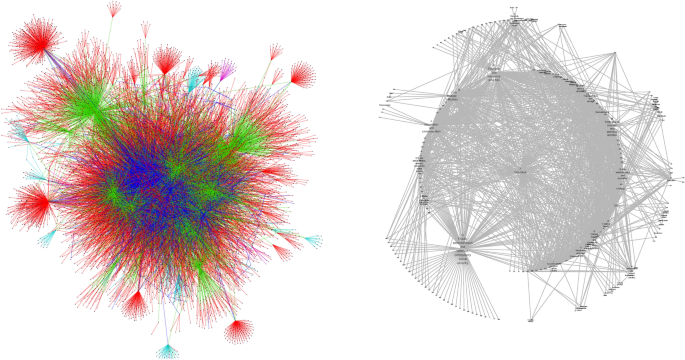The image features two distinctive renderings of abstract 3D objects set against a completely white background. On the right side, there's a minimalistic, grey-toned structure formed by interconnected points and lines, creating a spherical shape with random lines extending outward, giving it a skeletal appearance. On the left, a more intricate and colorful 3D object is depicted, composed of intertwining red, green, and blue lines that form a loosely spherical, organic shape with elements protruding from its center. The contrast between the simple, monochromatic structure on the right and the vibrant, complex form on the left highlights the diversity in the abstract artwork.